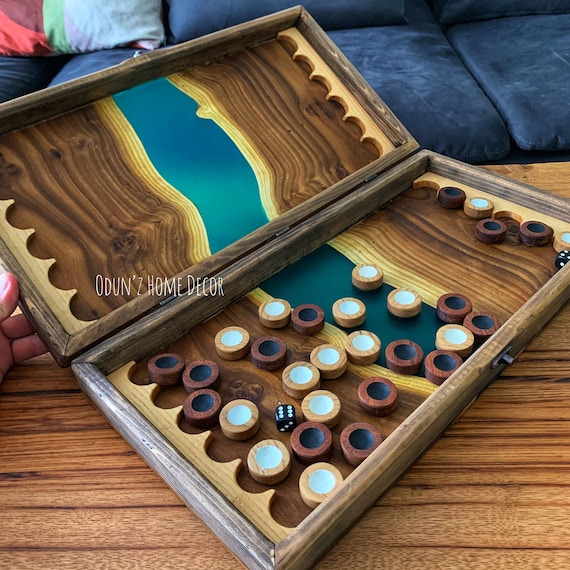In the image, we see an intricately designed wooden board game case, likely for a classic game such as Go or a similar variant. The case features an oak finish and is placed upon a mahogany cocktail table. The wooden box is open, revealing its contents: circular playing pieces organized into black and white sets. Each playing piece is rimmed, with the black ones showing cherry wood detailing and the white ones having a more natural, whitewashed rim. Centrally positioned inside the box are two black dice, one in the very center and the other in the top right corner.

The inner part of the case showcases a striking design: a deep blue line, accented with cyan and yellow, stretches horizontally across the middle, creating an impression of flowing water. This line continues seamlessly across the case's break where the hinges are. 

A hand is seen holding the top of the case open on the left side, though the hand itself is out of focus, making it difficult to identify the person. Behind the game, a plush, blue velvety couch is visible, providing a comfortable and luxurious backdrop. The couch is accompanied by colorful cushions in the top left of the image. At the bottom of the opened case, the brand name “Oh Dunn's Home Decor” is visible, hinting at the high-quality craftsmanship of the board game.